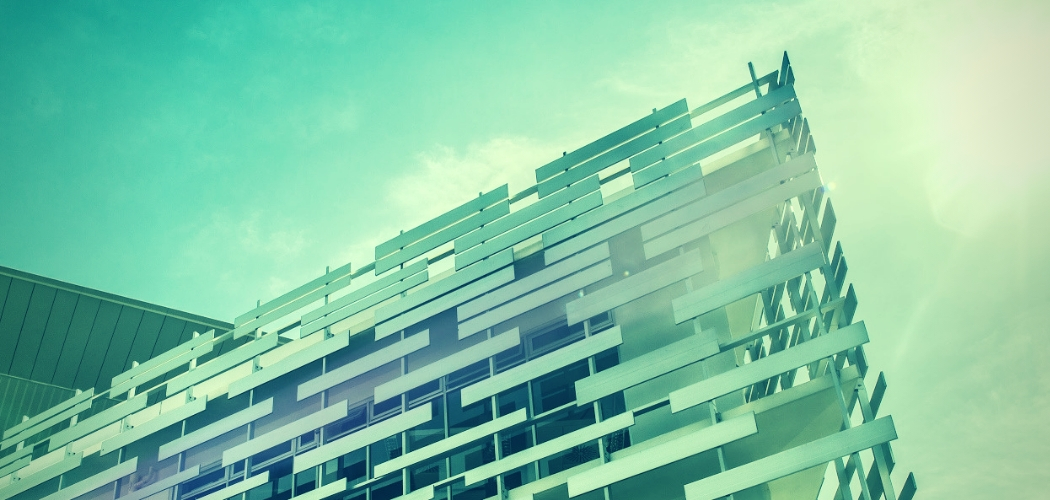The image showcases an incredibly innovative and bold exterior design of a building. The façade appears to be sheathed in a unique wall system, designed to allow air, light, and elements of nature to pass through its surface. The horizontal panels are strategically spaced apart, enabling the free flow of wind, light, and offering glimpses of the sky through the structure. This not only provides functional benefits but also contributes to an aesthetically pleasing and architecturally intriguing appearance. 

Of particular interest is where this wall meets the adjoining structure at the apex; the lines of the panels do not align perfectly. This staggered positioning suggests a creative, possibly AI-driven design process, hinting at the potential use of artificial intelligence in the architectural design. The juxtaposition of these meticulously positioned panels against a light green background and set against a backdrop of an overcast sky further enhances the visual appeal and complexity of the design. The asymmetry at the meeting point subtly indicates the innovative approach taken in materializing this architectural marvel.